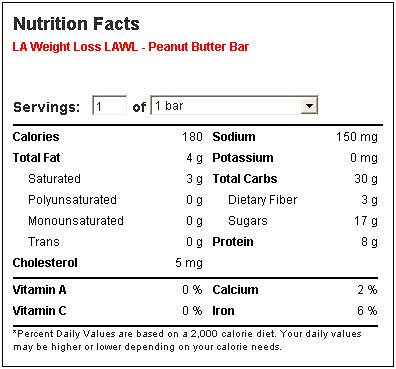The image depicts the Nutrition Facts label of an LA Weight Loss (LAWL) Peanut Butter Bar. The box is predominantly white with black trimming and black text, except for the product name which is written in red. The label is formatted into two main columns. The left column lists the contents in a hierarchical manner: "Calories 180, Total Fat 4 grams, Saturated Fat 3 grams, Polyunsaturated Fat 0 grams, Monounsaturated Fat 0 grams, Trans Fat 0 grams, Cholesterol 5 milligrams." The right column details: "Sodium 150 milligrams, Potassium 0 milligrams, Total Carbs 30 grams, Dietary Fiber 3 grams, Sugars 17 grams, Protein 8 grams." Below these columns, a dividing black line precedes information on vitamins and minerals: "Vitamin A 0%, Vitamin C 0%, Calcium 2%, Iron 6%." An additional black line clarifies that the "Percent daily values are based on a 2000 calorie diet. Your daily values may be higher or lower depending on your calorie needs." Overall, the clean and precise layout aims to provide comprehensive nutritional information at a glance.